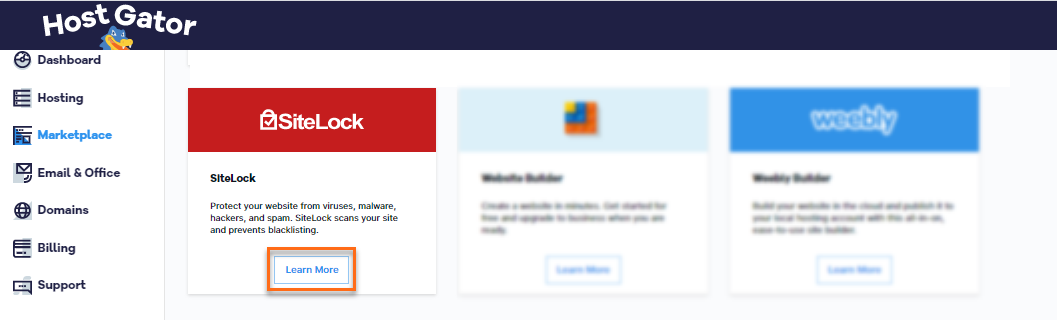This image is from the Host Gator program's website. At the very top, there is a long horizontal blue bar featuring the text "Host Gator" on the left. Beside the text, there is a small, cheerful cartoon of an alligator's head, rendered in blue and white, with an orange and yellow mouth.

On the left-hand side of the image, there is a vertical navigation menu containing several labeled options: 

1. **Dashboard** - Marked by a small circle icon.
2. **Hosting** - Indicated with a set of lines.
3. **Marketplace** - Represented by a box with lines.
4. **Email and Office** - Denoted with a box featuring a letter icon.
5. **Domains** - Symbolized by a globe icon.
6. **Billing** - Illustrated with an envelope icon.
7. **Support** - Depicted with a box containing three dots.

Prominently displayed to the right of the menu is a section with three selectable options, the first of which can be read clearly. It is labeled "SiteLock" with a red banner. Underneath, there is a description that reads: "SiteLock protects your website from viruses, malware, hackers, and spam. SiteLock scans your site and prevents blacklisting." Below this description, there is a button labeled "Learn More."

The remaining two options, "Website Builder" and "Weebly Builder," are partially visible but blurred, making their content unreadable. The faint colors hint at their presence, but no further details can be discerned from the image.